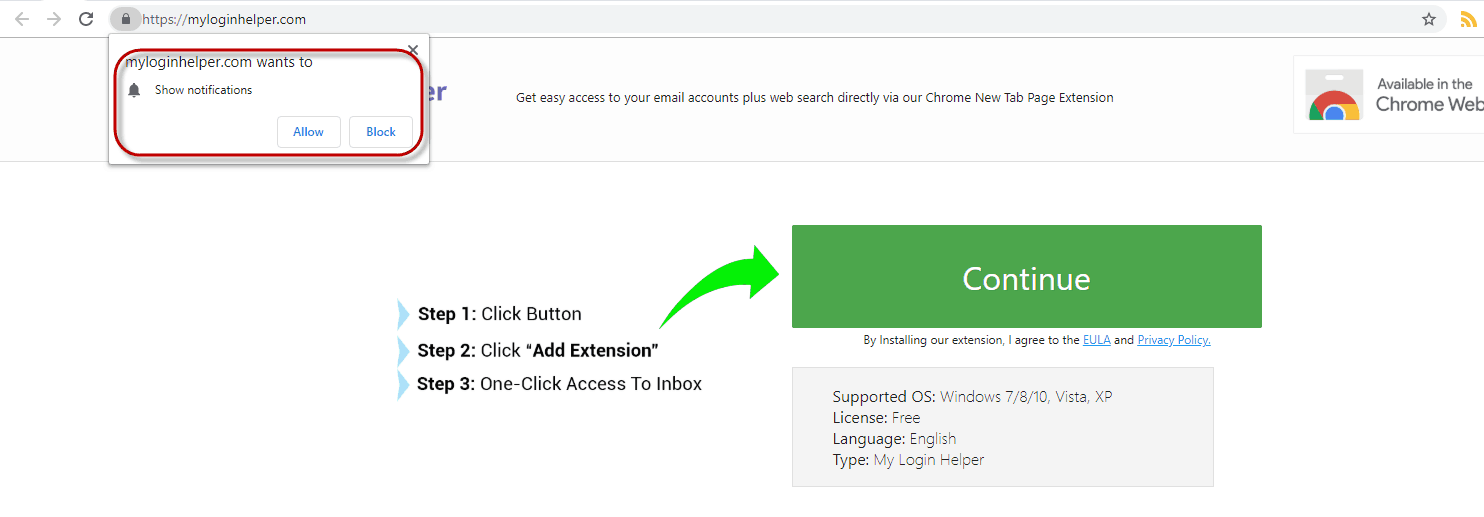The image appears to be a computer screenshot with a long rectangular layout, featuring a gray bar at the top. This bar displays a web address, "myloginhelper.com." Beneath this, there is a prominent white box encircled in red, which is a notification prompt stating, "myloginhelper.com wants to show notifications," accompanied by "Allow" and "Block" options on the bottom right, both outlined in blue.

To the right of this notification, a sentence reads, "Get easy access to your email accounts. Plus web search directly via our Chrome new tab page extension." At the upper right corner of the image, the recognizable Chrome symbol—a colorful circle—indicates the extension's availability, as it states, "Available in the Chrome Web Store."

Centered in the lower portion of the image, a large green rectangle contains the word "Continue" in white text, highlighted by a green arrow pointing towards it from the left. Adjacent to this green box, step-by-step instructions are provided: 
1. Click button 
2. Click add extension 
3. One click access to inbox."